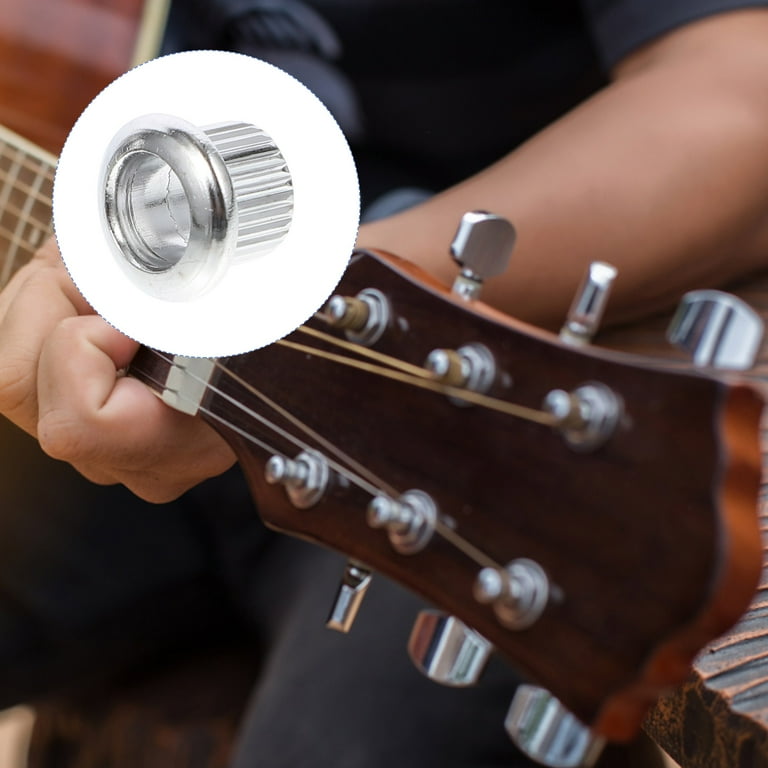The image is a full-color, digitally enhanced, posed photograph featuring a close-up view of a person playing an acoustic guitar. The overall image is square without any border or background. Prominently, in the upper left corner, a white circle has been superimposed, showcasing a round, silver metallic piece. This piece appears cylindrical with a hollow center and ridged sides, likely a part or accessory for the guitar. The hand of the player, identifiable by their Caucasian skin, is wrapped around the neck of the brown wooden acoustic guitar, forming a chord. The guitar's headstock is centered in the image, though only a small portion of the guitar’s body and neck are visible, and the player's blue jeans can be seen, but their top remains out of frame.